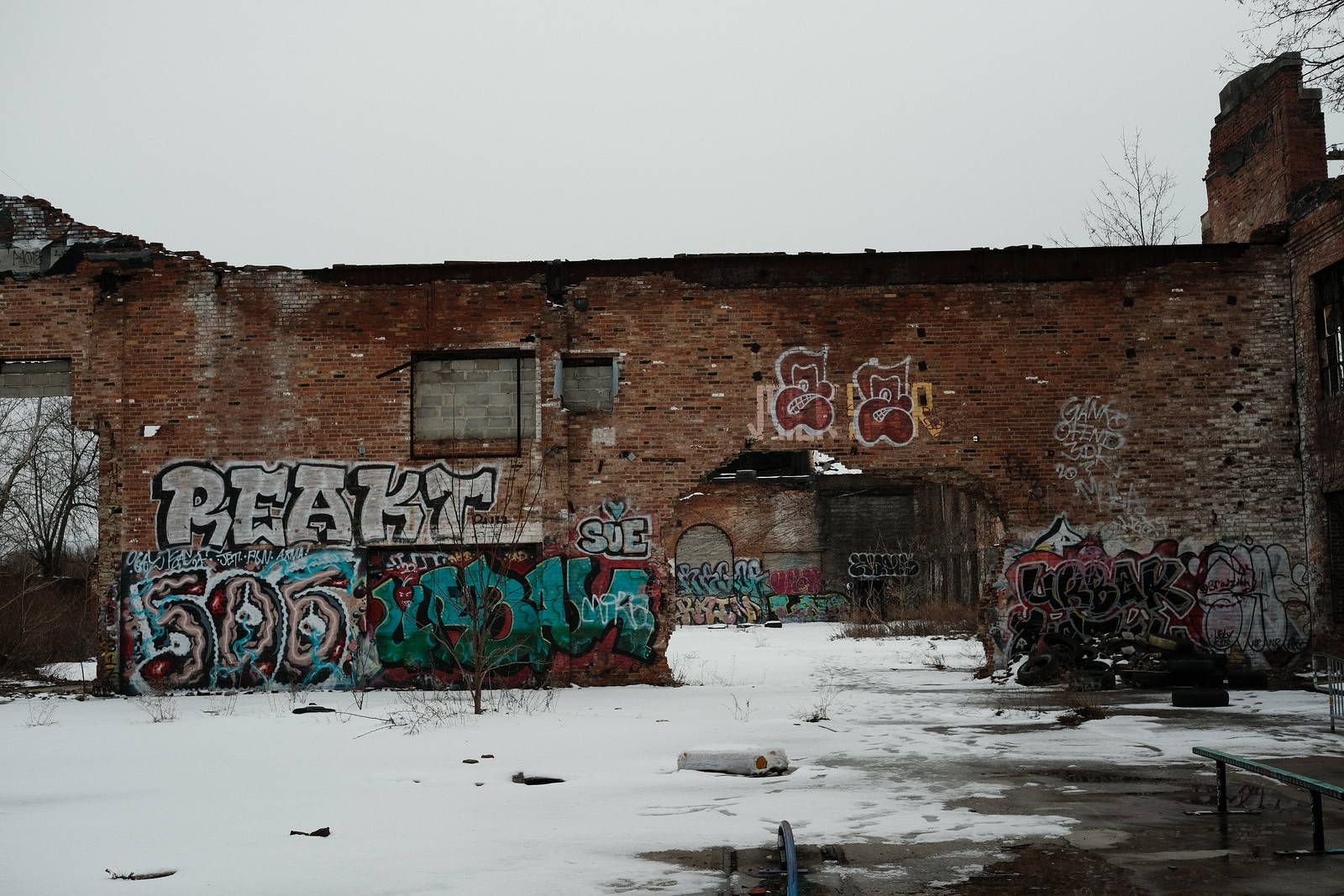The image depicts a derelict, dilapidated brick building set in a winter landscape with snow covering the ground and patches of slush visible in the bottom right corner. The brick wall in the foreground, tinged with red, features several large, gaping holes, possibly remnants of former garage doors. Smaller, bricked-up windows are interspersed throughout the structure. The wall boasts extensive graffiti, including words like "react," "5:05," and possibly "Erbeck," painted in various colors such as white, blue, and red. A small archway opening near the center leads to a courtyard area with additional walls adorned with graffiti. Visible through another gap in the wall, a leafless tree stands against an overcast, gray-white sky, adding to the abandoned, wintry ambiance of the scene. Guardrails are present in the bottom right corner, accentuating the and the deserted feel of the location.